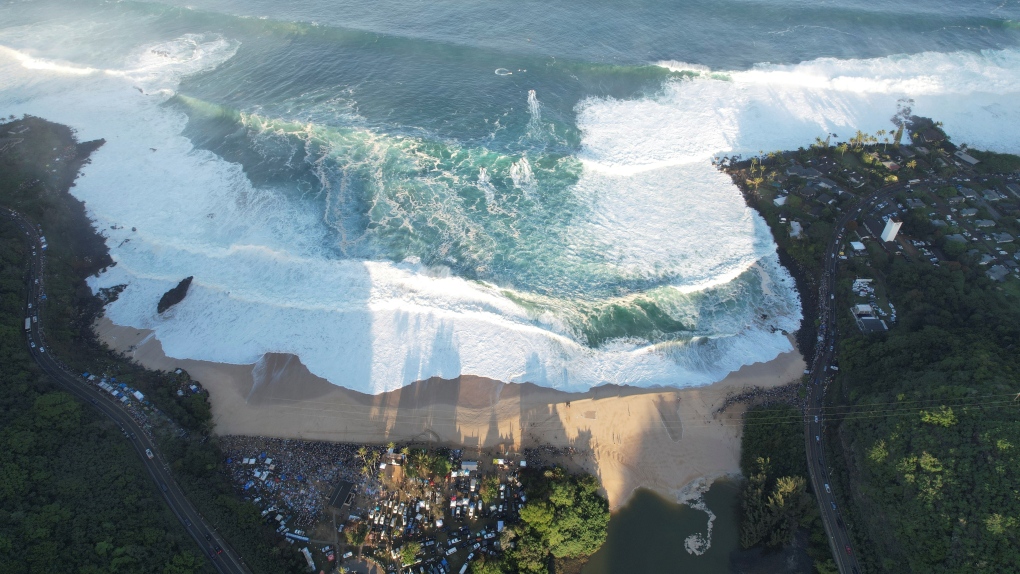The image is an aerial view of a coastal landscape, with the ocean's rough, white-capped waves crashing onto a sandy beach. The sea is a greenish-blue, and the waves appear exceptionally high and forceful, almost as if they are flooding the area. The shoreline curves into a cove, bordered by green shrubbery and a winding road that trails behind the beach. On the wide plateau to the right, and extending around the beach, there are numerous houses and vehicles, which look particularly small and vulnerable against the encroaching water. A rock juts out into the surf on the left side of the image, adding to the dramatic scene. Despite the absence of people, the sunlight casts long shadows, enhancing the vivid detail and giving depth to the landscape, reinforcing the view from above, likely captured by a drone or aircraft.